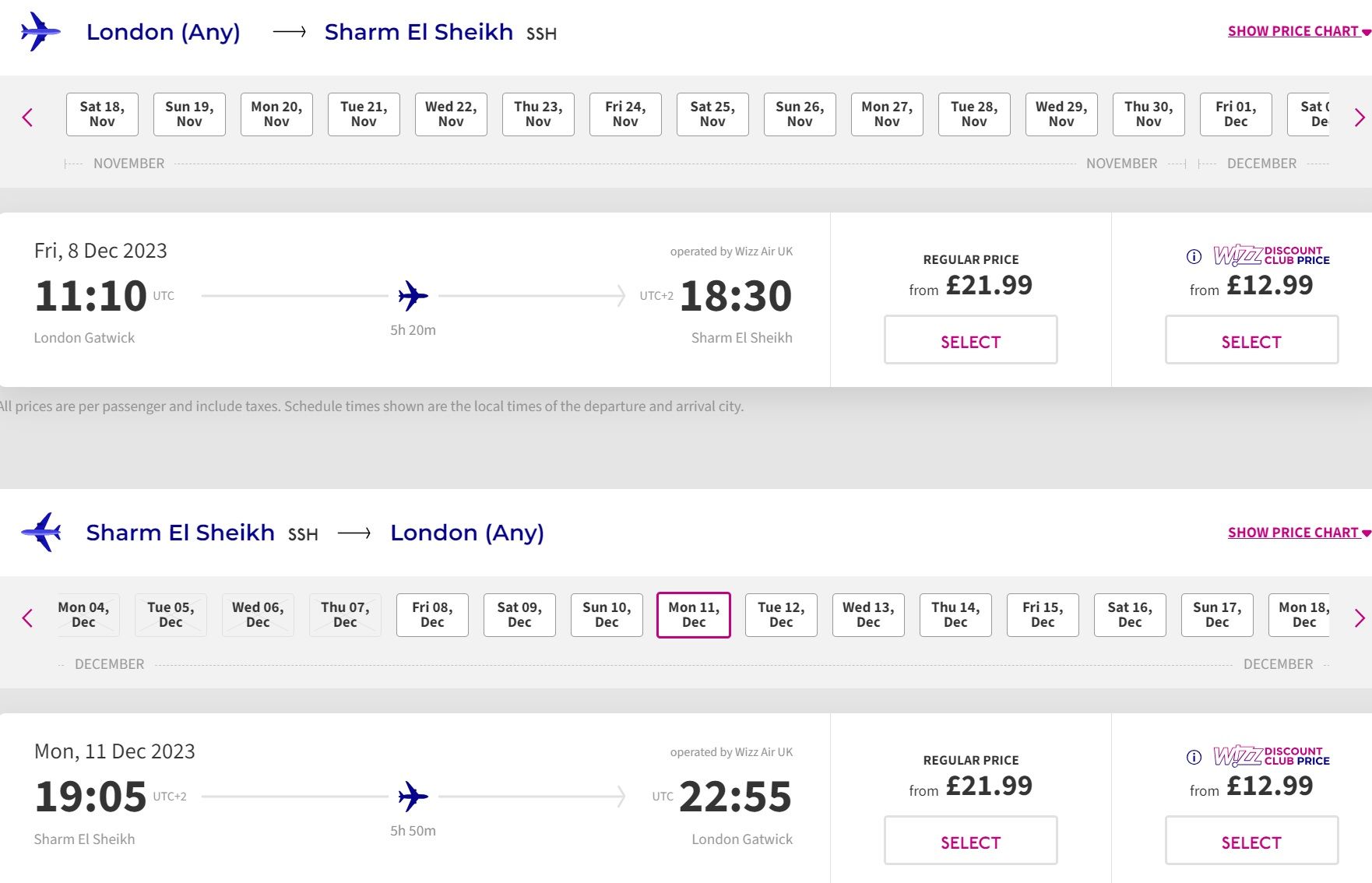The image displays a digital flight information screen.

In the top left corner, it shows the departure city "London". On the top right, the destination is listed as "Sharm El-Sheikh". Next to the destination, a price chart appears in purple font. 

Directly below the destination and price chart, a list of around a dozen selectable dates is visible, without specific times attached. 

Further down, detailed flight information is provided for a particular journey. The entry indicates a flight on Friday, 8 December 2023, departing at 11:10 and arriving at 18:30. To the right, the flight cost is prominently displayed: Regular fare at €21.99, with a pink "Select" button nearby, and a discounted fare at €12.99, also with a pink "Select" button below. 

A grey background section separates this information from the return flight details.

For the return journey, the selected date is Monday, 11 December 2023. The return flight departs Sharm El-Sheikh at 19:05 and lands back in London at 22:55. Similar to the outbound flight, the pricing options are displayed to the right with two fares and pink "Select" buttons.

This concludes the entirety of the information presented on the screen.